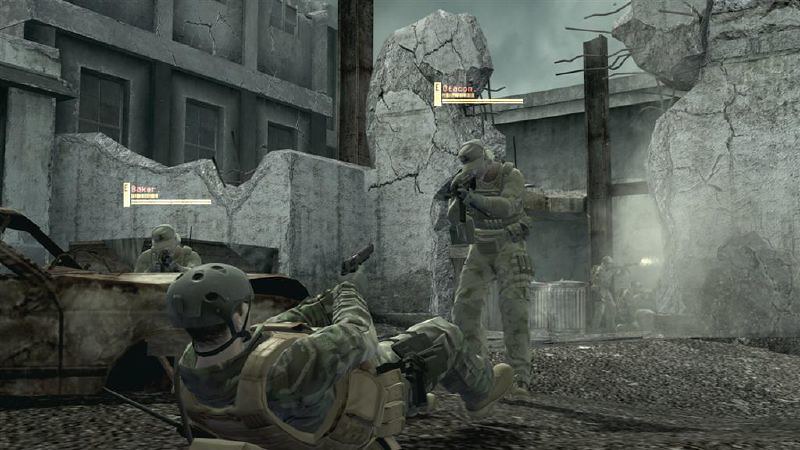The image appears to be a screenshot from a video game set in a war-torn cityscape. The environment is dominated by gray stone ruins, with twisted metal rebar jutting out from the debris, creating an atmosphere of desolation and destruction. On the left side of the scene, there is a burned-out car, adding to the apocalyptic setting. 

In the foreground, a dramatic confrontation unfolds: a man in green camouflage lies on his back, facing away from the camera, aiming a pistol upwards at another man. This second man, also in green camouflage, stands over him, facing the camera, pointing an assault rifle downwards at the man on the ground. 

Adding to the tension, a third man is partially obscured behind the burned-out car. He is crouched down and aiming his gun at the man lying on the ground. Both the standing man and the crouching man have life meters hovering above them, indicating their status as characters in the game.

In the background, other figures can be seen engaging in a firefight, their gunfire adding to the chaotic ambiance, although they are barely visible due to the smoke and rubble. The entire scene is a gritty depiction of urban warfare, caught in a frozen moment of intense conflict.